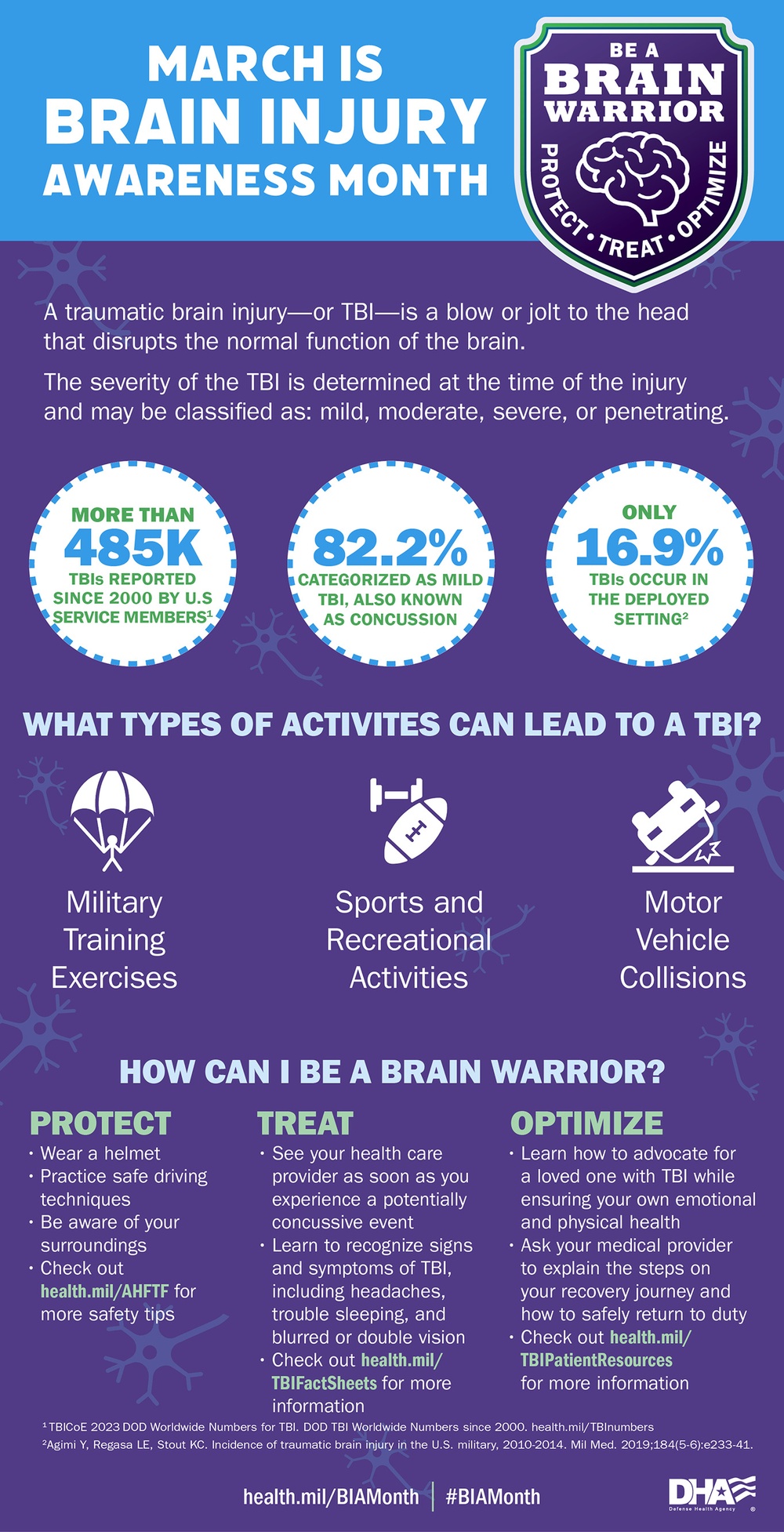This infographic, from the DHA, is a detailed poster predominantly in blue and purple that highlights Brain Injury Awareness Month. At the top, it reads in white text, "March is Brain Injury Awareness Month," and features an emblem to the right with "Be a Brain Warrior" inscribed inside a shield-like shape. The words "Protect, Treat, Optimize" encircle a line drawing of a brain within the emblem. The poster provides extensive information about traumatic brain injuries (TBI), emphasizing their impact and statistics. It defines a TBI as a blow or jolt to the head that disrupts brain function, with severity classified as mild, moderate, severe, or penetrating. Key statistics are highlighted in three white circles with blue-dotted outlines: more than 485,000 TBIs reported since 2000 by U.S. service members, 82.2% of which are mild TBIs or concussions, and only 16.9% occurring in deployed settings. The poster further details activities leading to TBIs, illustrated through images: military training exercises (parachute), sports and recreational activities (sports equipment), and motor vehicle collisions (overturned car). It concludes with actionable steps for being a "Brain Warrior," organized into three columns—Protect, Treat, and Optimize—each listing preventive and treatment tips to enhance brain health. The DHA emblem and a flag are also visible, reinforcing the poster's authoritative source.